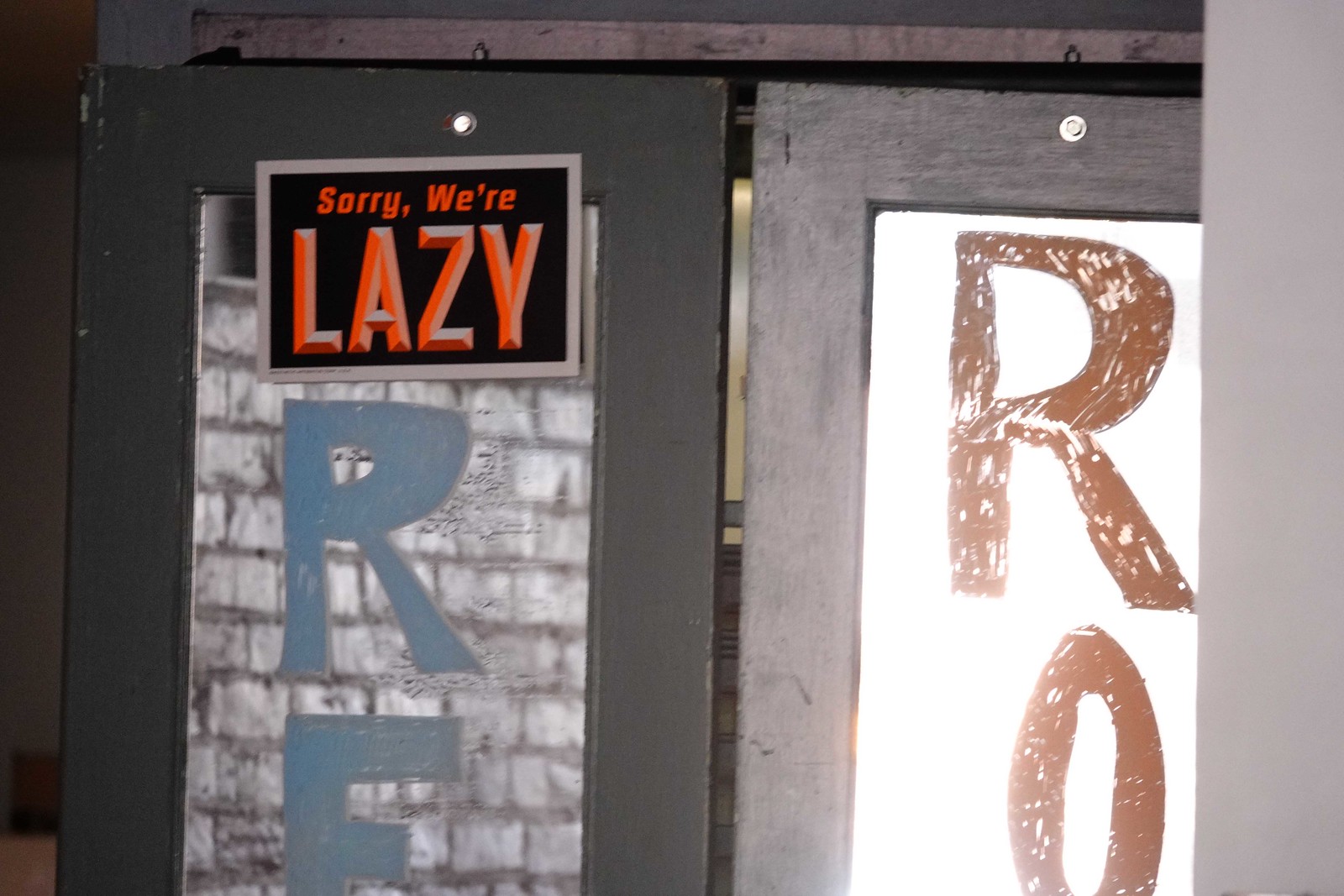This image appears to be taken indoors, showcasing the entrance or exit of a restaurant or bar with saloon-style double doors. The doors open to the left and right, and are made of wood. On the left door, there's a window that appears to be mirrored, reflecting a brick wall. The window features the letters "RE" in light blue, handwritten style, and also shows some scratches and spots. There is a small circular mirror or pinhole at the top center of the left door. Additionally, a black sign with a gray border hangs on the left door with orange text that says "Sorry, We're," and below it, in large, 3D block letters, "Lazy" in red. This sign mimics the style typically used for "Sorry, We're Closed" signs. 

On the right door, there is a light gray outer border and another small mirror or pinhole at the top center. The central part is painted white, possibly replacing old glass. The white surface features the letters "RO" written in red. The combination of these details suggests a creative and perhaps humorous environment, where imperfections and playful signage are part of the decor.